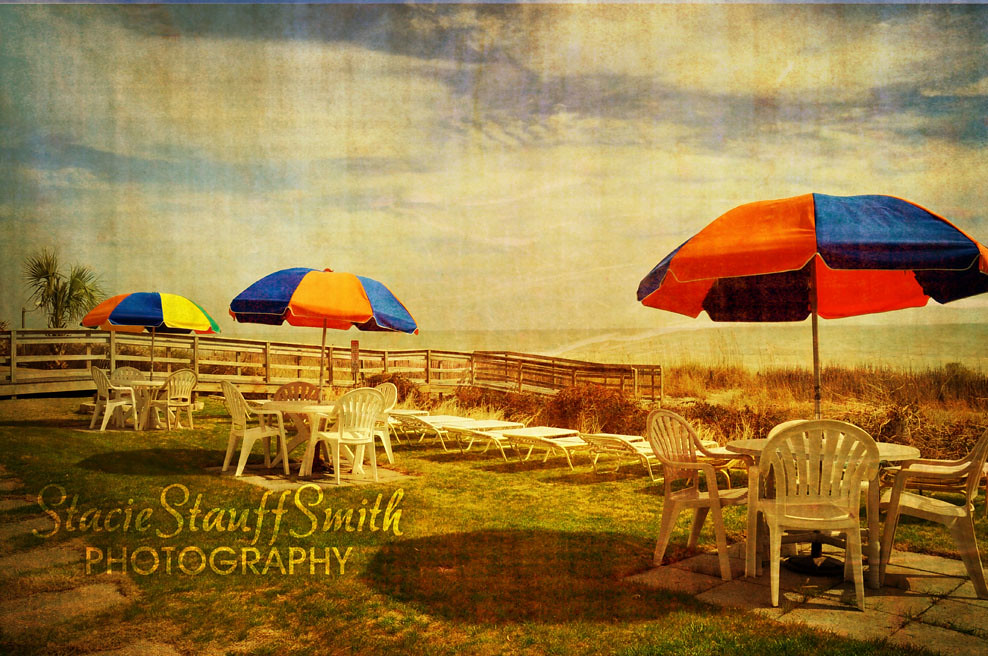This seemingly vintage and sepia-toned photograph, marked with the watermark "Stacey Stoff Smith Photography" at the bottom, captures a picturesque coastal scene. The image, framed with a photorealistic and fabric-like texture, presents a serene, bright day under a sky adorned with wispy, white clouds. The foreground features a grassy field scattered with sparse patches and a boardwalk-like pathway on the left. Nestled within this grassy area are three tables, each surrounded by four white, plastic chairs arranged around rectangular concrete blocks. Each table is sheltered by a multicolored umbrella, displaying vibrant hues of orange, blue, yellow, red, and green. Situated behind this setup are several lounge chairs aligned neatly. The background showcases a tropical palm tree on the left side, leading towards a distant view of the ocean, hinted at by the sandy beach and blurred landmass beyond. The photograph exudes an old-fashioned charm, possibly reminiscent of a vintage postcard, complete with visible creases that add to its nostalgic allure.